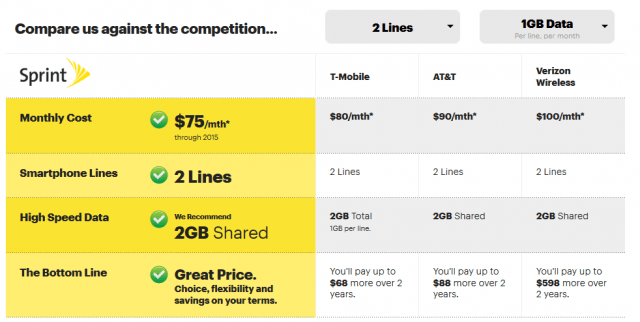The rectangular image, approximately five inches wide and two inches high, is split into two sections: left and right. The left side features a white header with black text stating "Compare us against the competition." Below the header, there are two gray rectangles with text; the first reads “two lines” and the second “one gigabyte data per line per month.” Beneath these, the left-hand side lists details about Sprint's offerings with a white background: monthly cost starts at $75 for two lines, with two gigabytes of shared high-speed data. At the bottom, it boasts "The bottom line: great price, choice, flexibility, and savings on your items."

The right-hand side is divided into three columns comparing Sprint with T-Mobile, AT&T, and Verizon. Each carrier’s monthly cost for two lines is displayed: T-Mobile at $80, AT&T at $90, and Verizon at $100, all for two gigabytes of data. Additionally, it states the long-term cost differences, indicating that with T-Mobile, customers would pay up to $68 more over two years, with AT&T up to $88 more, and with Verizon up to $598 more compared to Sprint.